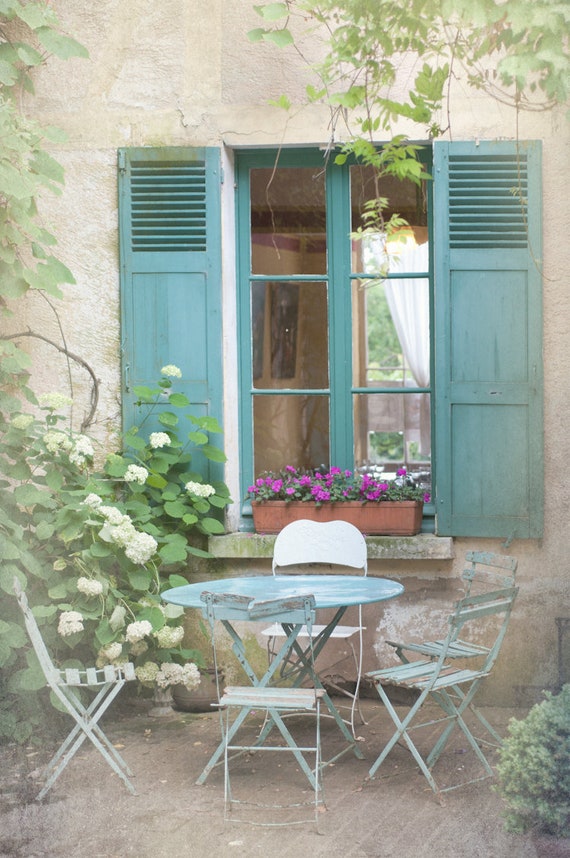This photograph captures a quaint outdoor scene in front of a stone house with a beige, rough-textured wall. The focal point is a long vertical window with blue-green shutters and a sill adorned with a brown rectangular pot containing vibrant fuchsia flowers and green leaves. The windowsill is weathered, displaying patches of green and brown moss. Inside the window, partially visible, are white curtains and hints of another room with brown walls and pictures.

In the foreground is a circular blue metal table surrounded by five chairs, including four rusty, light bluish-gray wooden chairs and one white metal chair. The seating arrangement rests on a gray brick surface, adding to the rustic ambience. To the left, a green bush with white flowers adds a touch of nature, while additional green creeper plants and vines cascade from the top left corner, enhancing the overall charming and slightly overgrown look of this serene outdoor setting.